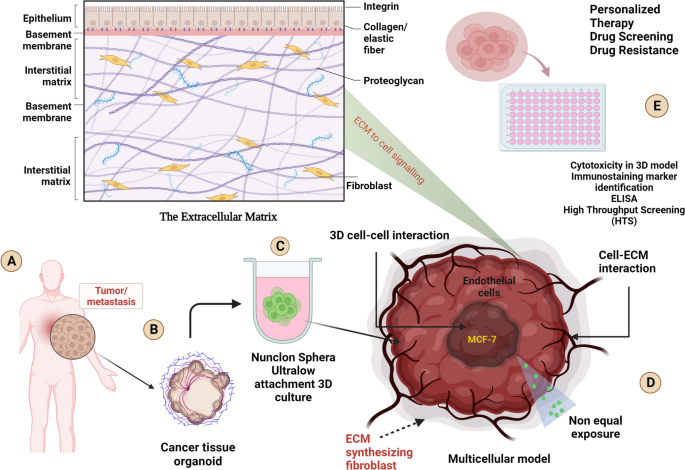A highly detailed anatomical illustration showcasing various components and interactions within a tissue environment:

- **Left Section:**
  - **Rectangle:** Displays purplish, wavy lines, situated against a yellow background.
  - **Organism-like Structures:** Yellow elongated organisms with a darker circle at their centers.
  - **Epithelium (Top Label):** Includes blue squiggly worm-like illustrations.
  - **Integrin and Collagen/Elastic Fiber (Right Labels):** Positioned adjacent to the epithelium.
  - **Basement Membrane:** A pinkish layer with interspersed purple dots.
  - **Interstitial Matrix (Left Label):** Located beneath the basement membrane.
  - **Proteoglycan (Right Label):** Corresponds to the interstitial matrix.
  - **Another Basement Membrane:** Potentially marking the end or a different section.
  - **Fibroblast (Right Label):** Positioned beneath another section labeled interstitial membrane.
  - **Extracellular Matrix (ECM):** Illustrated as a green area connecting to a bottom right diagram, resembling a brain.

- **Right Section (Bottom Right Brain-Like Diagram):**
  - **ECM to Cell Signaling:** Labeled in red against a green background.
  - **Endothelial Cells (Left):** Part of the diagram.
  - **MCF-7:** Highlighted in yellow within a central darker blob.
  - **3D Cell-Cell Interaction (Left Label):** Located near the bottom left.
  - **ECM Synthesizing Fibroblasts:** Labeled in the bottom left corner.
  - **Multicellular Model:** Written directly beneath in black letters.
  - **Non-Equal Exposure (Right Label):** Another section with green dots leading to a blue background.
  - **Step D:** Indicated by a black "D" wrapped in beige, marking the fourth step in this broader process.
  - **Cell ECM Interaction:** Noted at the top right.

- **Top Right Sequences:**
  - **Step A:**
    - **Tumor/Metastasis:** Cells in a circular formation with red markers indicating cancer on a person.
  - **Step B:**
    - **Cancer Tissue Organoid:** Depicted by a blue blob with a darker brown center, featuring pinkish and beige areas.
    - Arrow leads to…
  - **Step C:**
    - **Nucleon Sphera Ultra-Low Attachment 3D Culture:** Looks like a test tube containing pink liquid and green cells.
  - **Step D:**
    - **3D Cell-to-Cell Interaction:** Leading up to the extracellular matrix, as previously detailed.
  - **Circle with Pink Cells:** Transitioning to a blue rectangle filled with pink cells.

- **Step E:**
  - **Cytotoxicity in 3D Model:** Involving immunostaining marker identification, ELISA, and high-throughput screening (HDS).
  - **Personalized Therapy (Top Right):** Covers areas of drug screening and drug resistance.

This comprehensive diagram explicates various cellular interactions, tissue structures, and model steps, ultimately illustrating detailed processes crucial to understanding cancer dynamics and potential therapeutic pathways.